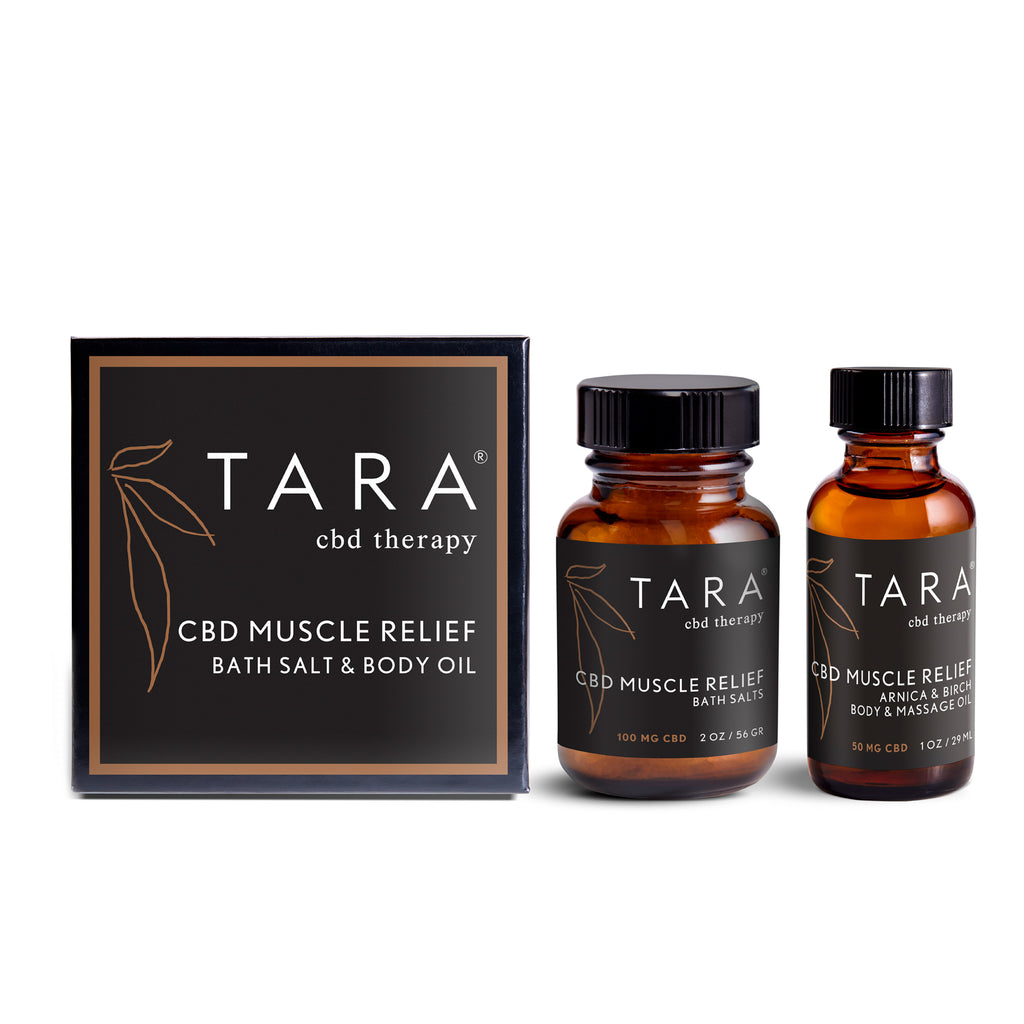The image showcases a set of CBD muscle relief products against a clean, white background. On the left side, there is a black rectangular box with a smaller brown rectangle inside it. Inside the brown rectangle, white letters spell out "Terra CBD Therapy" prominently, with the TERRA being uppercase and larger. Below, in smaller white letters, it reads "CBD Muscle Relief Bath Salt and Body Oil." The logo, which features a leafy design, is also present in bronze. On the right side of the image, there are two brown glass bottles with black screw tops. Each bottle has a black label with white text. The bottle on the left is labeled "Terra CBD Therapy, CBD Muscle Relief Bath Salts, 100 mg," indicating a net weight of two ounces or 56 grams. The thinner bottle on the right is labeled "Terra CBD Therapy, CBD Muscle Relief Arnica and Birch Body and Massage Oil, 150 mg CBD."